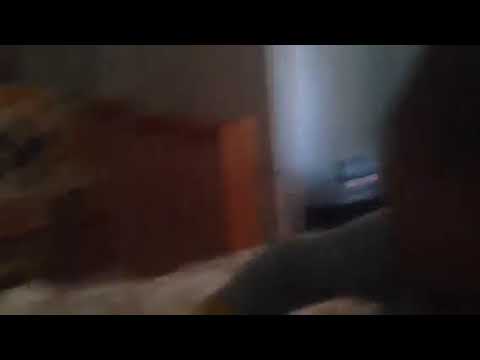The photograph is extremely blurry and grainy, making it difficult to discern specific details. The image appears to be taken indoors, possibly in a room with various objects and furniture. In the center-left of the photo, there's a brownish-red shape that resembles a bookshelf or small shelving unit. The immediate foreground features a greenish object, while the right side displays a dark, backlit shape that could be part of someone's head or body. A white door is faintly visible in the very center of the image. The overall picture is in a letterbox format with black borders at the top and bottom, suggesting it might have been taken in motion. The background to the center-right seems to show some clothes or sheets stacked on a black bin. The photo's pixelation and poor quality render most elements indistinct, resulting in a chaotic mix of colors and shapes, difficult to interpret with certainty.